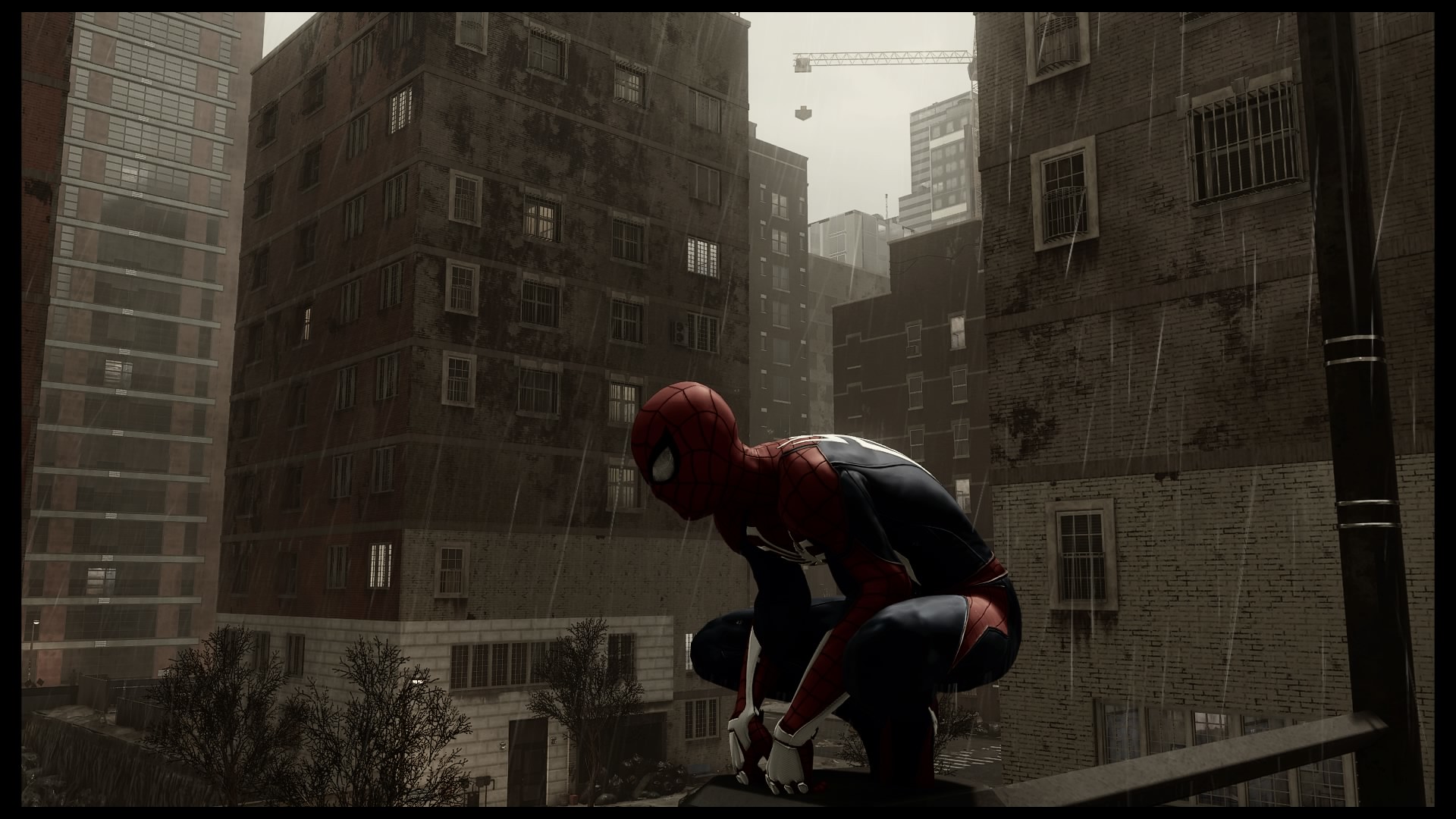The image depicts a detailed CGI rendering of Spider-Man perched on the railing of a balcony, viewed from the side. He is wearing his iconic red and blue suit, complete with white accents on his gloves and a white spider emblem on his chest and back. Spider-Man is crouched, with his face turned to the left, and his arms resting between his knees. The scene is set in a rainy, overcast cityscape, adding a dim and dreary ambiance to the image. 

In the background, several tall buildings can be seen: a prominent brick building to the left, a modern glass and concrete structure further left, and a rectangular building with numerous windows in the middle. At the top right of the screen, a tall crane is visible, indicating ongoing construction work in the distant background. The lower left corner of the image reveals the tops of trees below, likely part of an urban courtyard. Raindrops are falling across the scene, emphasizing the dreariness and adding texture to the atmospheric setting.